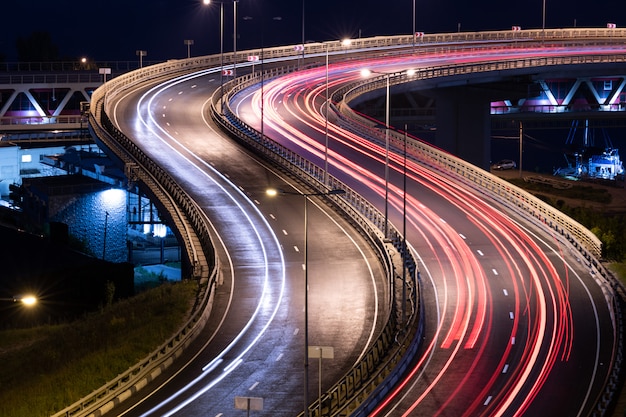This is a highly detailed, long-exposure photograph of an elevated, curved stretch of highway at night, showcasing an array of intricate light trails. The highway, captured from a lofty vantage point, demonstrates a sweeping S-shape, starting at the bottom left corner and twisting upwards to the top right. The left-hand side of the highway is adorned with continuous white ribbons of light created by the headlights of oncoming vehicles, while the right side features red streaks from the taillights of cars moving away, with hints of pink and gold.

Streetlights illuminate the highway, revealing its elevated structure, possibly passing over a body of water or a dock, with what appears to be buildings or warehouses beneath. The background suggests a mix of industrial and residential areas, with faintly glowing lights indicating other structures, perhaps a bridge, neighborhoods, or even billboards. Additionally, a railway line runs parallel in the background, also elevated and faintly lit.

The highway itself comprises four lanes, divided by a central barrier equipped with further lighting. The setting is predominantly dark, accentuating the brilliant light trails that dominate the image, creating a vibrant, almost surreal spectacle against the night sky.